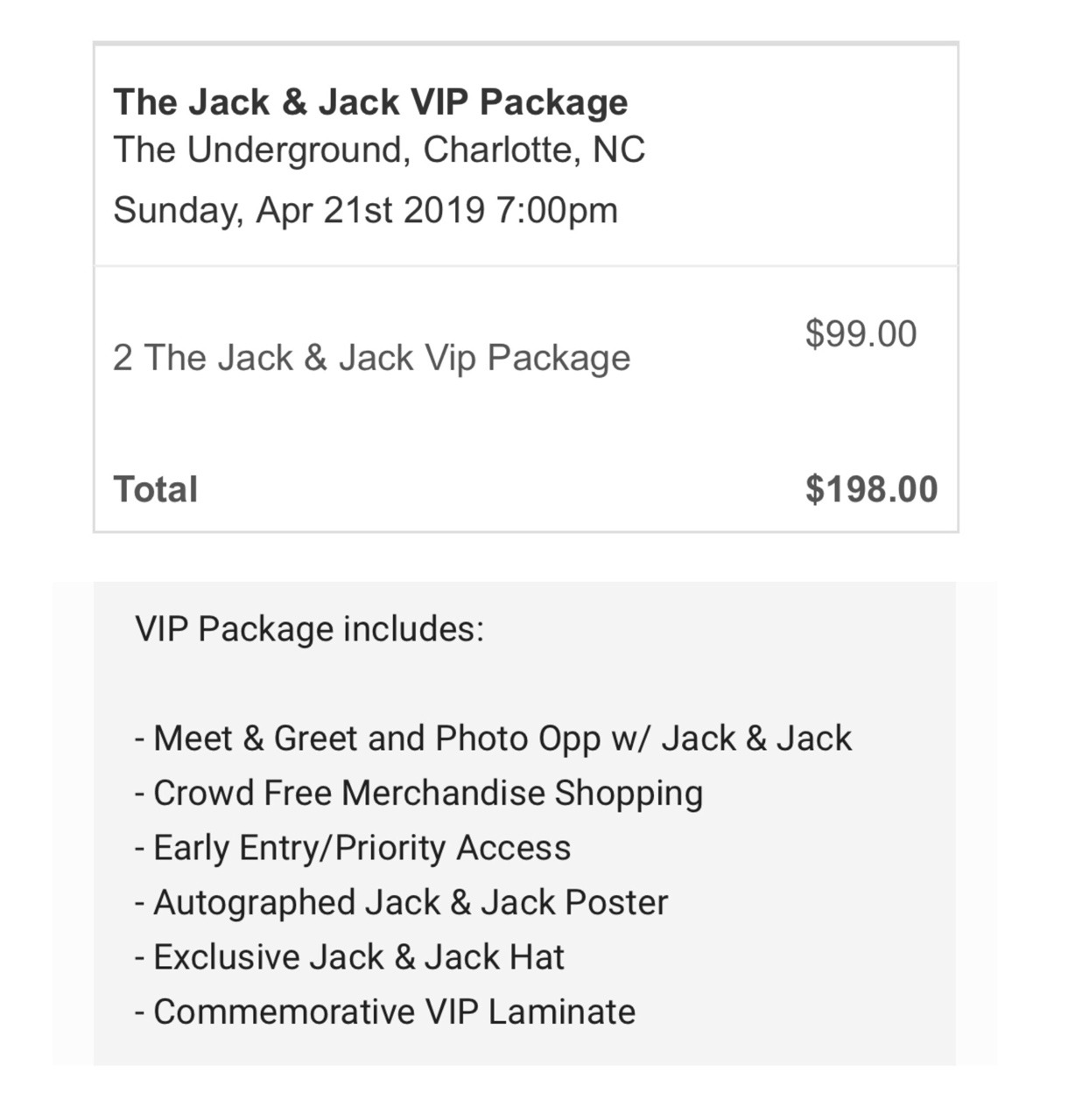The image showcases an order confirmation or receipt with details of a VIP package purchase. The layout features two distinct sections.

The first section is a rectangular box with a thin gray border and a white background. In the top left corner, bold black font reads "Jack and Jack VIP Package." Below this, in less bolded black font, it states "The Underground in Charlotte, North Carolina." The date and time are provided underneath: "Sunday, April 21st, 2019, 7pm." A thin gray line runs beneath this information, separating it from the next area. In this lower section, the left side indicates "Qty: 2" for the Jack and Jack VIP package, while the right side displays the price as "$99.00" per package. At the bottom left corner, bold black font states "Total," with the figure "$198.00" in bold on the bottom right corner.

The second section sports a solid gray rectangular box. At the top left, in black font, it reads "VIP package includes:" followed by a list of included perks, each preceded by a dash. The list details:
- Meet and greet and photo op with Jack and Jack
- Crowd-free merchandise shopping
- Early entry priority access
- Autographed Jack and Jack poster
- Exclusive Jack and Jack hat
- Commemorative VIP laminate

This structured layout clearly presents the details of the VIP package purchase and benefits.